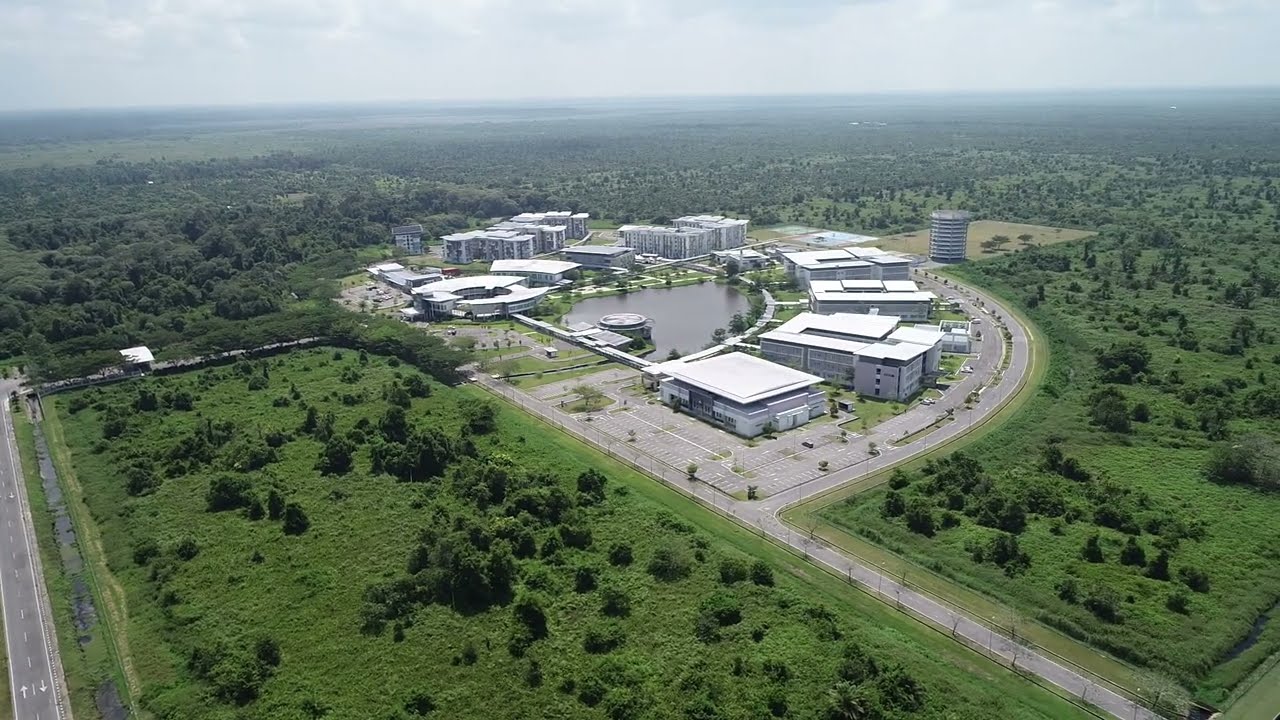This aerial image showcases a large commercial office park situated in a lush, green, rural area. The office park is uniquely shaped, resembling a quarter-circle or a half-diamond, with buildings organized along the outer edge and around a central pond. These structures, predominantly white and gray with flat roofs, vary in height from one to three stories, with some even taller, including a distinctive circular cylinder tower on the right side. Pathways and roadways encircle the complex, connecting the various buildings. The streets leading to the office park feature white lines and dashed markings, with two primary entrances visible at the bottom left. Surrounding the office park is a dense expanse of green vegetation, possibly a forest or woods, extending into the distance. In the center of the office park, there is a dark, still pond, adding to the serene environment. The sky above is a combination of blue with hazy white clouds, contributing to the tranquil rural setting. The overall region is abundant with greenery, enhancing the picturesque and peaceful ambiance of the office complex.